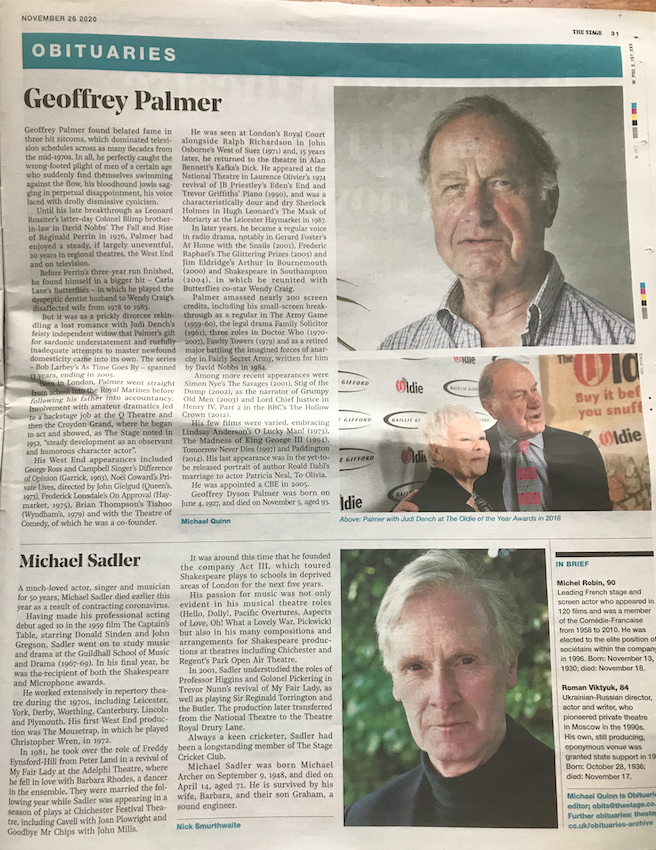This page, dated November 26, 2020, from "The Stage" newspaper, page 31, features two prominent obituaries with photographs. The top obituary memorializes Jeffrey Palmer. A distinguished older man, Palmer is pictured twice: in the top photo, he is alone wearing a checkered shirt; in the second, he is seen with actress Judi Dench at the Oldie of the Year Awards in 2018. The obituary describes Palmer's rise to prominence through three hit sitcoms spanning from the mid-1970s, capturing the essence of his signature roles portraying men facing life's unexpected challenges, marked by his distinctive, disappointed expression and a voice tinged with cynical joviality.

The second obituary on the page honors Michael Sadler, another elderly gentleman depicted in a headshot against a backdrop of greenery, dressed in black. Sadler is remembered as a beloved actor, singer, and musician whose career spanned 50 years. His obituary mentions his death earlier this year due to contracting coronavirus.

Additionally, on the right side of the page are brief obituaries for Michael, Michelle Robin, and Roman, providing a concise tribute to their lives and contributions.